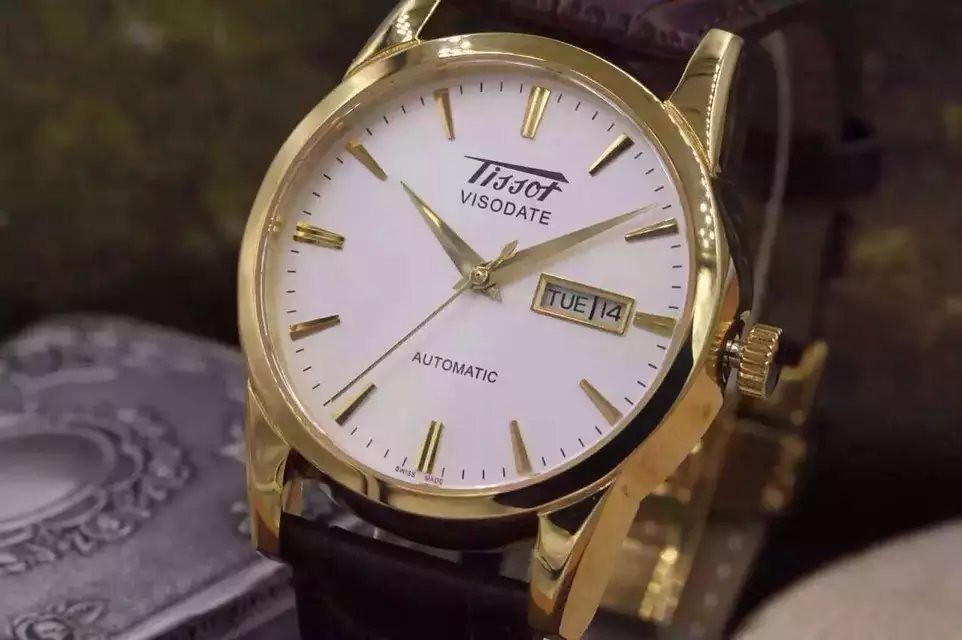This elegant wristwatch, crafted by Tissot, boasts a captivating white face adorned with gold bars that represent each numeral. The brand name "Tissot" is prominently displayed below the 12 o'clock position, followed by the model name "Visodate". Beneath the central pivot point of the clock hands, the word "Automatic" is inscribed, indicating the watch's self-winding mechanism. The hour, minute, and second hands are all fashioned in gold, matching the refined aesthetic of the timepiece. Positioned to the right of the watch’s center is a small window displaying the day and date, which currently reads "Tuesday the 14th." This window is framed in an elegant pewter color, adding a subtle contrast to the design. The watch's stem, used for setting the time and date, is also in gold, completing the harmonious and luxurious look of this sophisticated accessory.